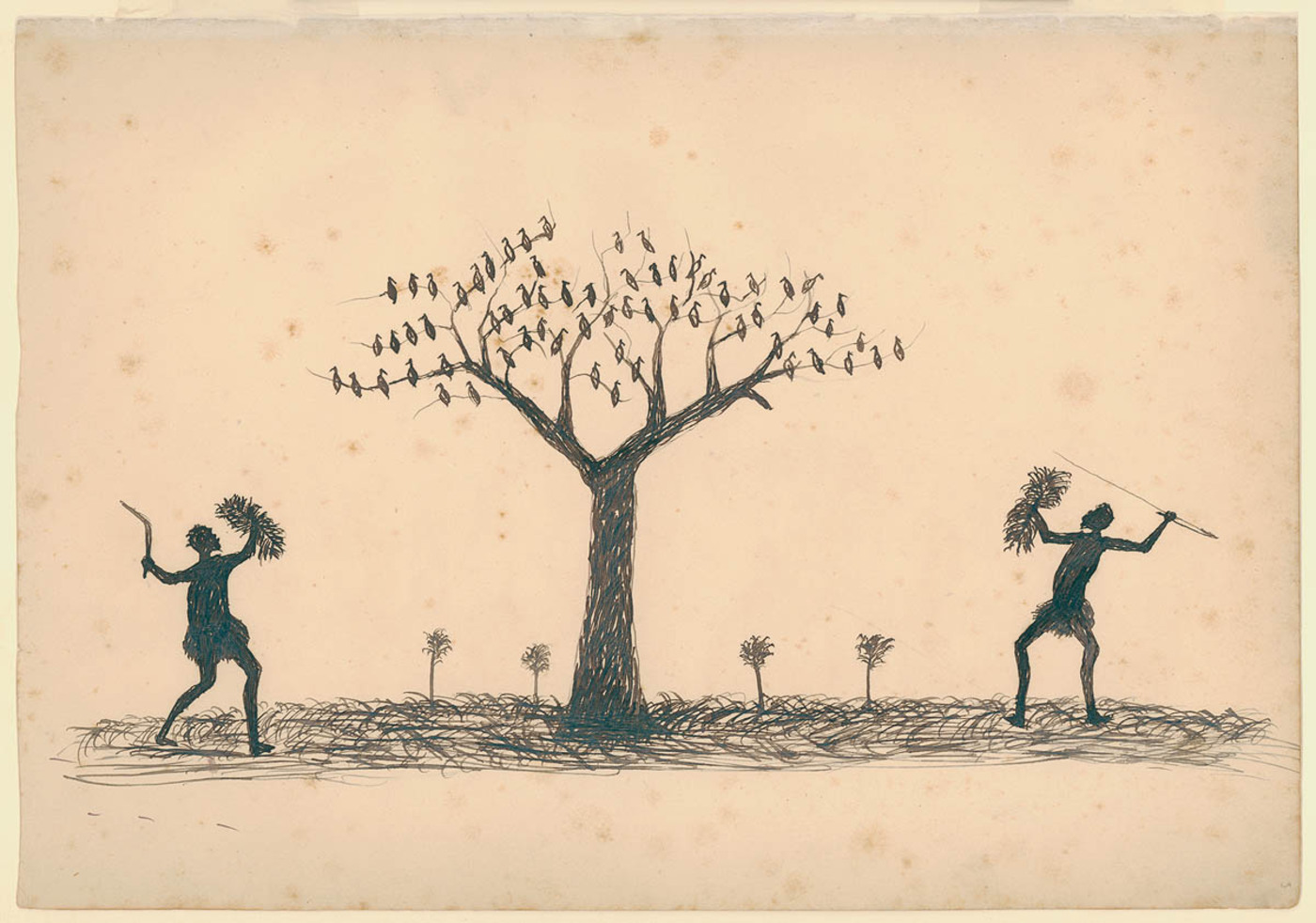This black and white line drawing depicts a scene of two tribal men engaged in hunting activities around a tall, leafless tree teeming with birds. The tree, characterized by a thick, dense trunk that branches out into very thin limbs, is a central element of the composition. Approximately 60 to 70 birds are scattered across the branches, which extend about 10 feet from the main split of the trunk. The ground beneath the tree is textured with black scribbles, suggesting a rough terrain, and is flanked by knee-high plants on either side.

The tribal men, positioned to the left and right of the tree, hold traditional hunting weapons; one clutches a spear while the other holds a boomerang. Each man also has a shield crafted from plants. Additionally, they are each carrying some form of brush or foliage, potentially straw or grass, in their other hands. Their postures and the direction of their weapons suggest an attempt to drive the birds out of the tree or to hunt them directly. The overall scene is rendered in a simple yet evocative black pen or pencil style, emphasizing the stark and fervent activity around the bird-laden tree.